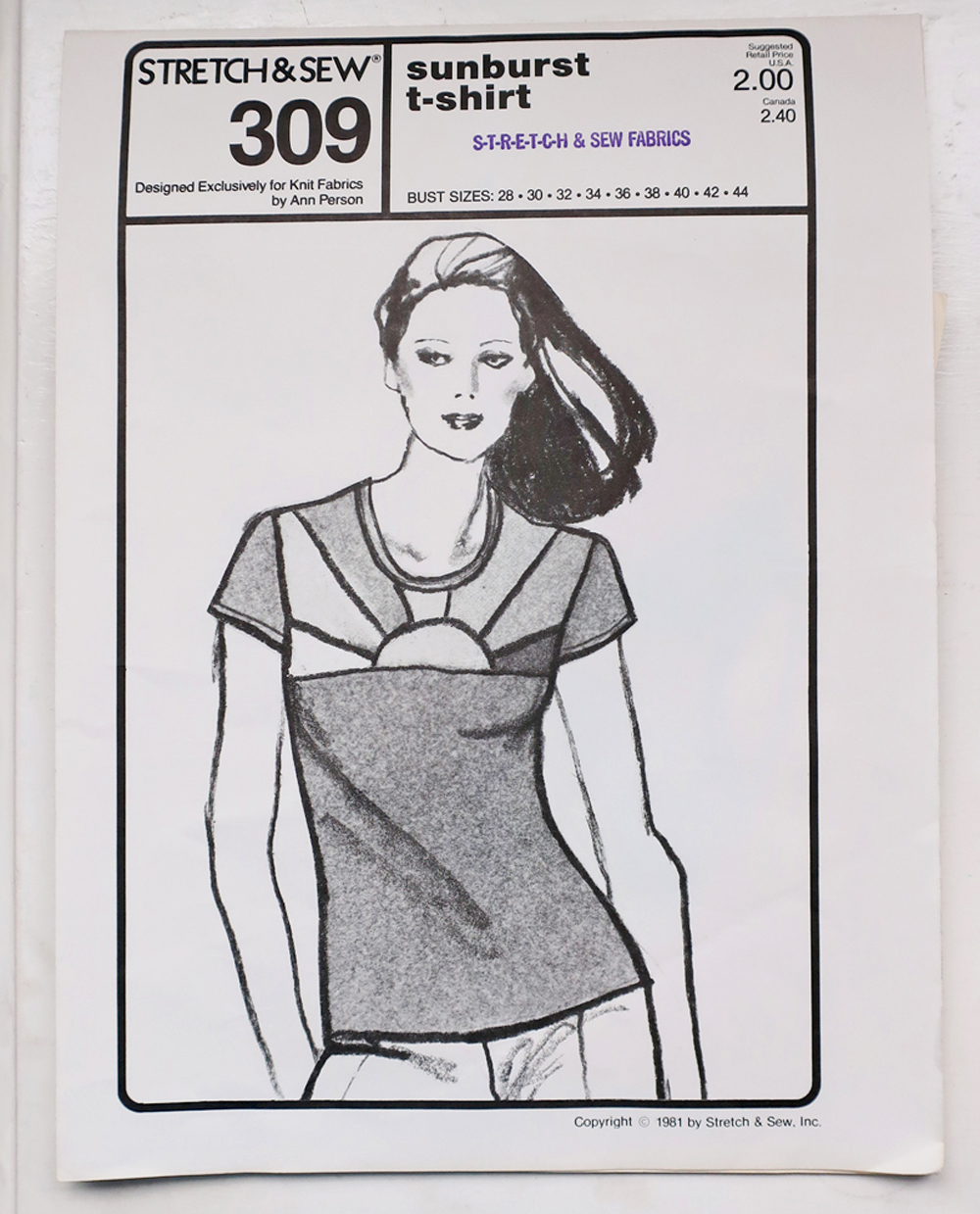This vertically aligned, vintage sewing packet features a detailed, black-and-white design. Set against a white background, the packet is bordered by a black frame. At the top, a small rectangular section outlined in black reads "STRETCH AND SEW" in all caps, followed by "309" in bold numbers. Below this, the text "Designed exclusively for knit fabrics by Ann Person" is displayed. To the right, within a longer rectangular section with a black border, the words "Sunburst T-shirt" are left-aligned. Stamped across the middle in blue letters is "S-T-R-E-T-C-H and sew fabrics." 

Dominating the center of the packet is a large, black-and-white line art illustration of a smiling woman with long dark hair cascading to her right side. She wears a short-sleeve t-shirt adorned with a sunburst pattern, featuring a half-circle and radiant lines emanating from the chest up to the neck area. The packet highlights various bust sizes, ranging from 28 to 44, listed at the bottom of the rectangular section. In the upper right-hand corner, the suggested postal prices are noted: $2.00 for the USA and $2.40 for Canada. Additionally, the lower part of the image is a grayscale representation, enhancing the vintage aesthetic of this classic print publication package design.